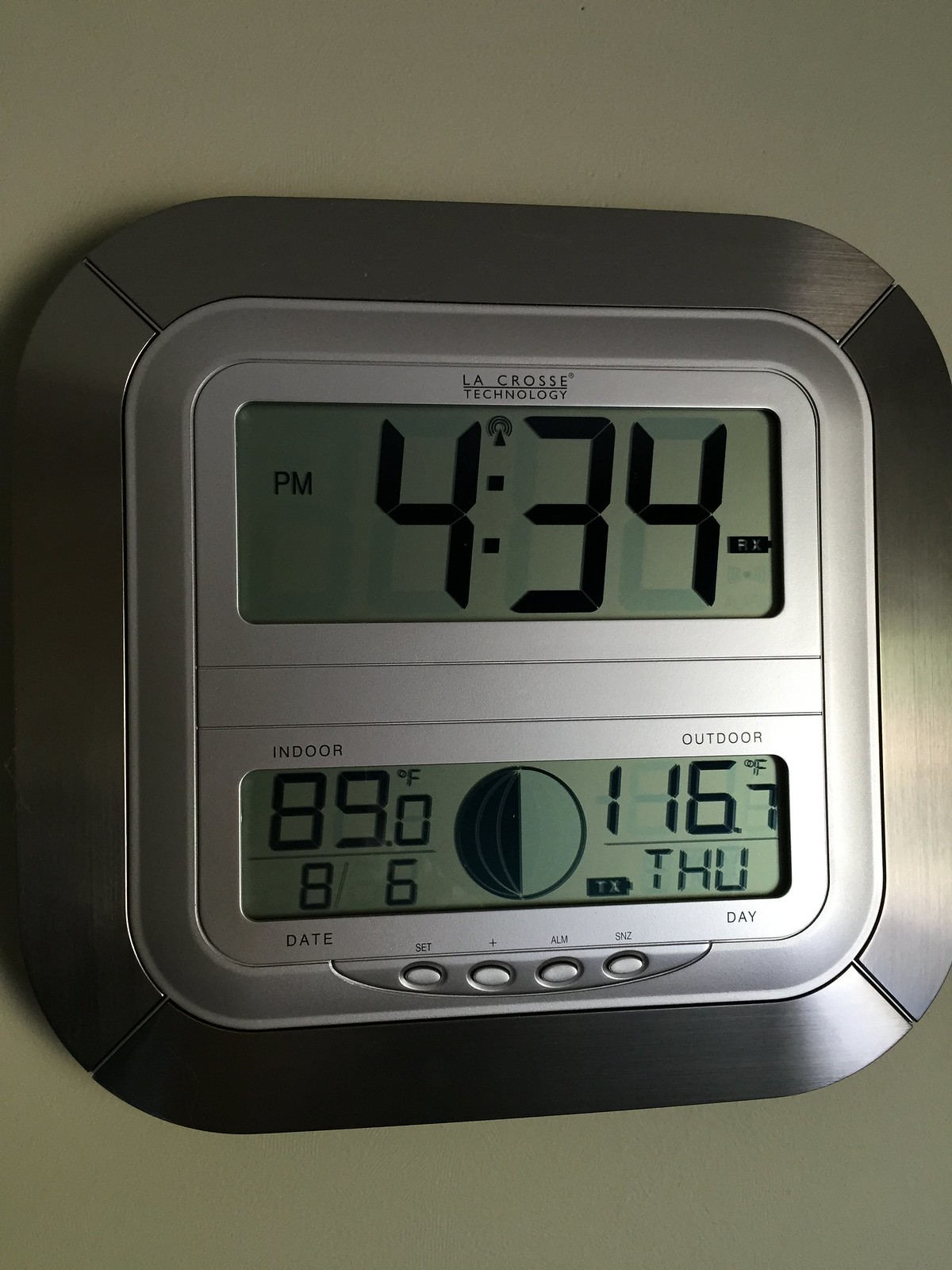The image features a close-up view of a wall-mounted device. The device appears to be a multifunctional digital unit that likely serves as both a thermostat and an alarm clock. It carries the brand name "La Crosse Technology," which is printed in small letters just above the display of the time.

The device is encased in a silver metallic mount, with its edges having a darker, shiny metallic finish. It is mounted against a light olive-green painted wall, providing a contrasting backdrop that highlights the device.

The unit has two distinct display sections:

1. **Top Display Panel:** 
   - Orientation: Landscape
   - Information displayed: 
     - Time: "4:33 PM"
     - Additional indicators: "PM" on the left
   - Interface: Digital Clock

2. **Bottom Display Panel:**
   - Orientation: Landscape
   - Information displayed:
     - Temperature: 
       - "Indoor: 89.0°F"
       - "Outdoor: 116.7°F"
     - Date: "8.6"
     - Day: "Thursday" abbreviated as "THU"
     - Additional symbol: A half-blacked-out circle (possibly indicating a moon phase)
   - Interface: Dual Thermostat and Calendar

Below the bottom interface, there are four small oval-shaped buttons aligned horizontally:
- The leftmost button is labeled "SET."
- The remaining three buttons have unclear or unreadable labels but likely serve various settings and adjustments purposes.

Overall, the wall-mounted device is a sophisticated gadget combining timekeeping, temperature monitoring (both indoor and outdoor), and date/day display features, with a potential additional function highlighted by the half-blacked-out circle symbol.